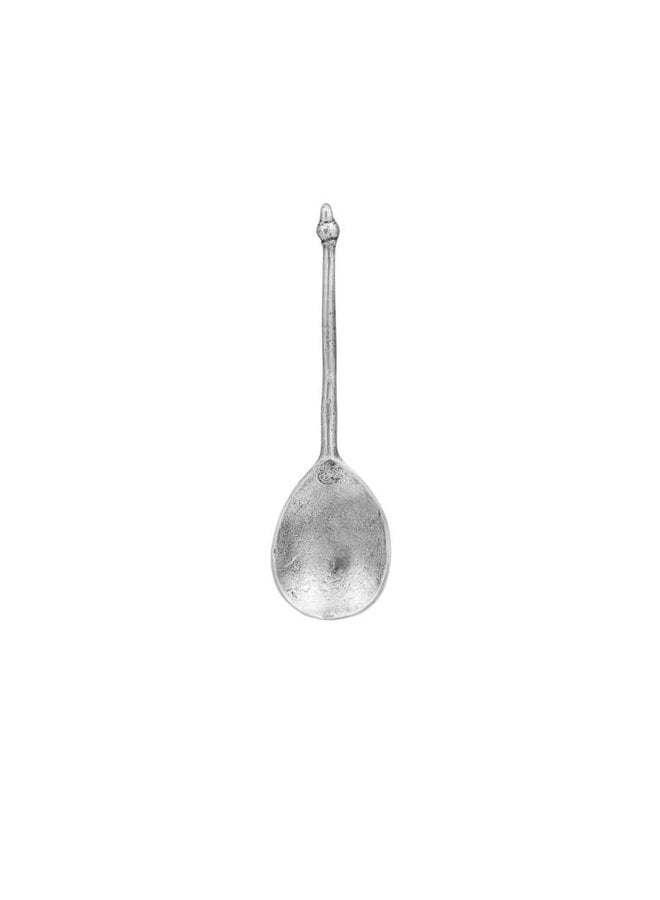This photograph depicts a lone, metallic spoon set against a stark white background. The spoon appears to be made of silver or potentially pewter or stainless steel. The handle is positioned vertically at the top of the image, with a dark silver line running through its middle, narrowing towards a slight bulbous tip. The spoon's stem is ribbed and thin, contributing to its elegant appearance.

The bowl of the spoon, situated at the bottom, is oval and portrayed from the convex side, suggesting we are looking at the back of the spoon rather than its concave front. The surface of the spoon is subtly rough, not entirely smooth, with a distinguishable smudge or varying reflection near the center of the bowl, likely caused by external lighting. The light source appears to be illuminating the lower part of the bowl, highlighting its contoured and slightly imperfect texture. The simplicity of the white background ensures that the intricacies of the spoon remain the focal point of the image.